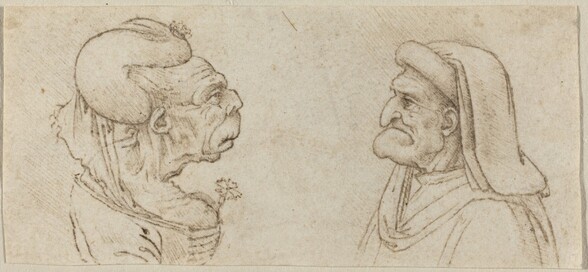This is an intricate line drawing resembling a vintage sketch, rendered in shades of brown on a pale, off-white background. It features two figures in a close exchange. On the right is an elderly figure, potentially a woman, with distinguishable wrinkles, a pronounced hooked nose, and a large chin, draped in a gown-like robe with a cowl around the neck. This figure wears a head cover that extends into a veil. On the left is an intriguing character with a broad nose, downturned ears, and lips, which gives it a semi-animalistic appearance, reminiscent of a dog or ape, yet it retains some human features. This figure has a flower prominently placed near the bust area, adding an element of curiosity. The background consists of melded white with dark paint marks, enhancing the focus on the exchange between the two figures, seemingly engrossed in a deep and silent conversation.